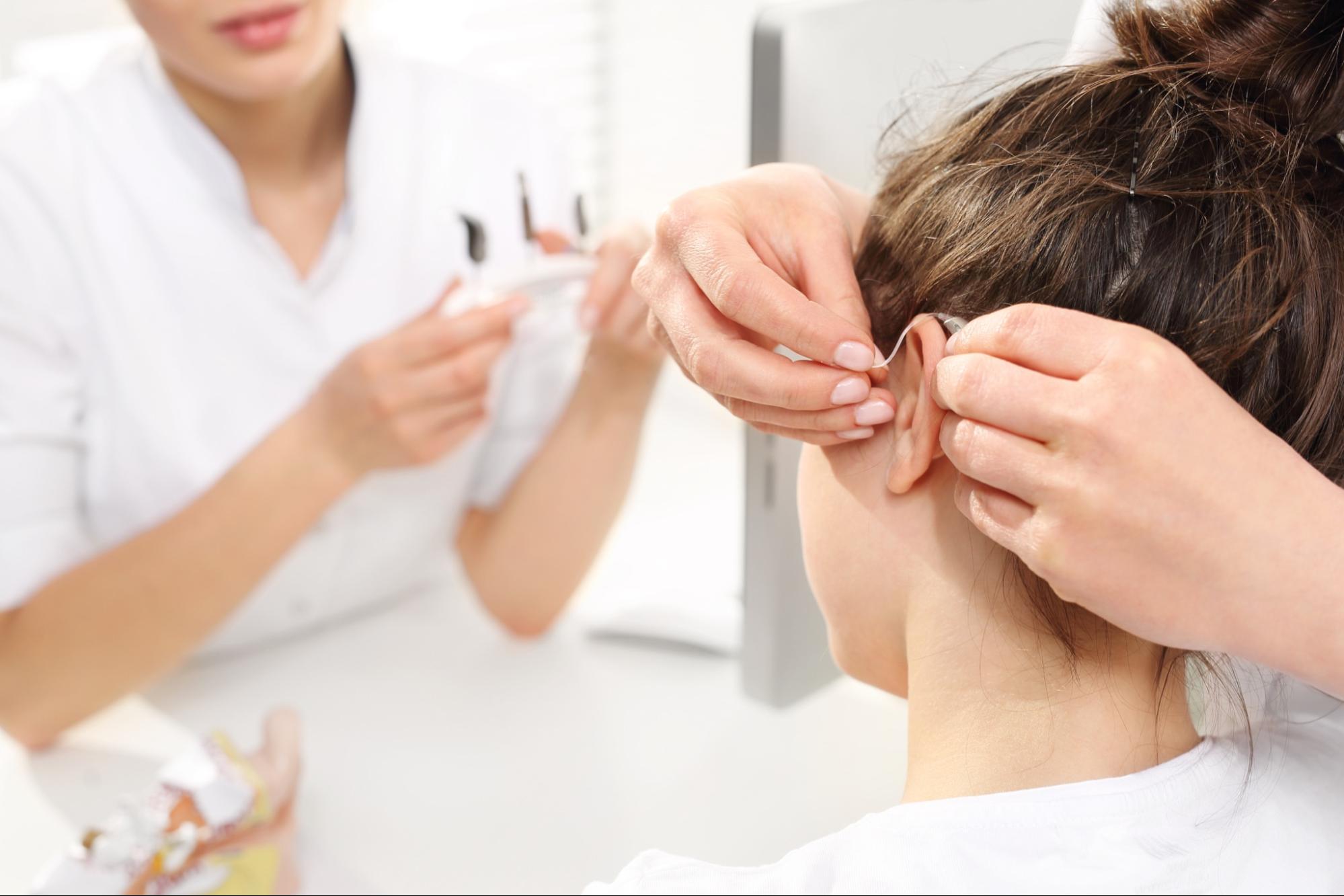This photograph captures a detailed, clinical setting where a young girl with brown hair is being fitted for a hearing aid or cochlear implant. The focal point of the image is the back of the girl's head, specifically her left ear, where two white hands—likely belonging to a medical professional—are carefully positioning the device. The device appears to wrap around the back of her ear, and part of it is being inserted into her ear canal. Both individuals in the image are white, and the professional, dressed in white, appears to be female. In the blurred background on the left, another woman, also in white and partially visible only from her lips down, is holding an indistinct object while resting her elbows against a counter. The clinical environment suggests a professional procedure, reminiscent of images found in medical brochures or pamphlets promoting hearing aid products. The colors in the image include brown, olive, white, gray, yellow, and pink.